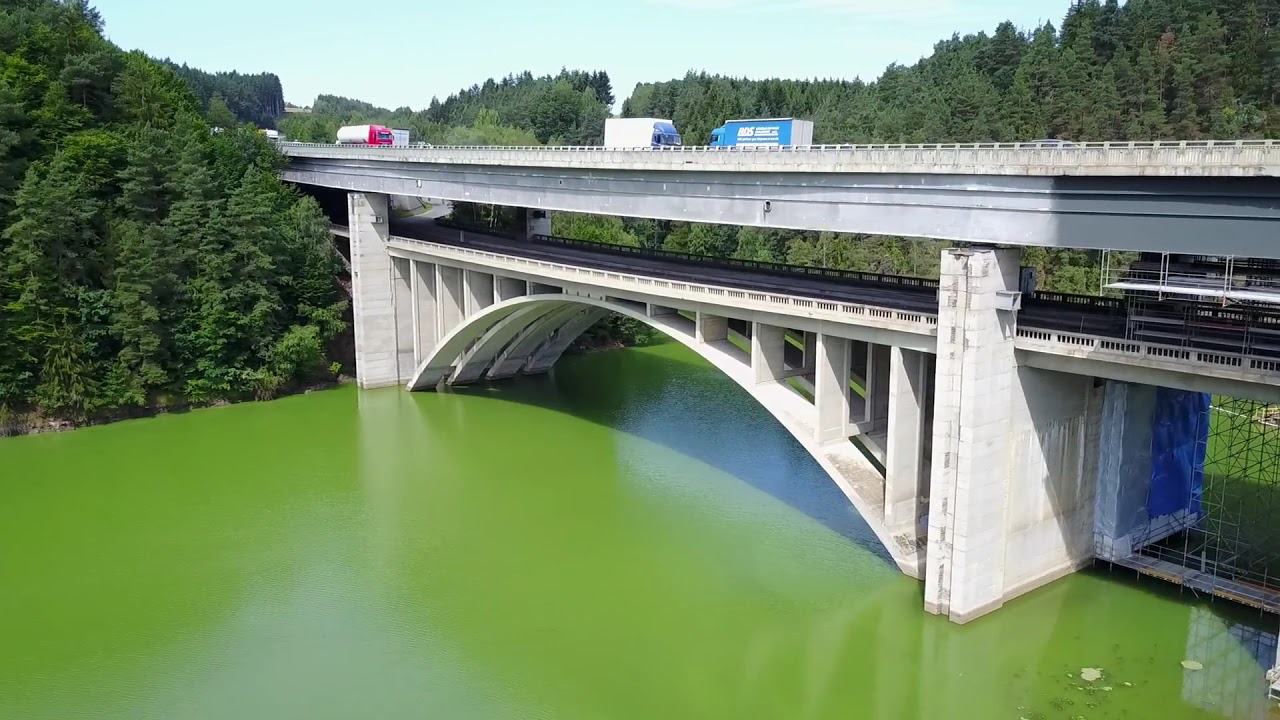The image depicts a large, concrete bridge spanning a green, algae-colored body of water, captured at a roughly 45-degree angle. The bridge features two solid, white brick columns with gray stains, extending from the water to support the structure. Between these columns is a curved archway, with the roadway situated above it. This roadway, under a very dark shadow, has barriers on both sides. Above this level is a second roadway with white barriers, upon which three trucks are visible. Traveling from left to right, there’s a truck with a red cab and a white trailer, a white box truck with a blue cab, and another box truck with a light blue cab and design. In the bottom right corner of the image, there’s a notable buildup of darker green algae. The background features a forest of lush, green trees on steep mountains, beneath a slightly hazy sky.